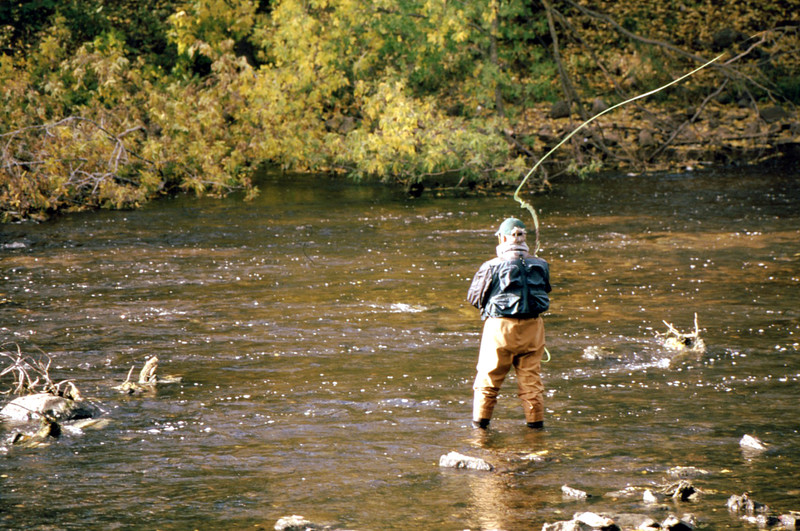The scene captures an elderly white male fly-fishing in a shallow, murky brown pond or river, surrounded by shrubbery and greenery. He stands ankle-deep in the water, clad in a light blue fishing vest, khaki pants, and black shoes. His gray hair is partially concealed by a blue baseball cap as he faces away from the camera, mid-cast with his fishing line whipping through the upper right portion of the image. The fisherman also wears a long-sleeved shirt and waders, and his dark green vest is equipped with multiple pockets. Around him, large boulders, smaller rocks, and branch debris lie scattered in the water's lower right and left corners. The background is composed of dense vegetation where the waterline meets the shore, with no other people or boats in sight.